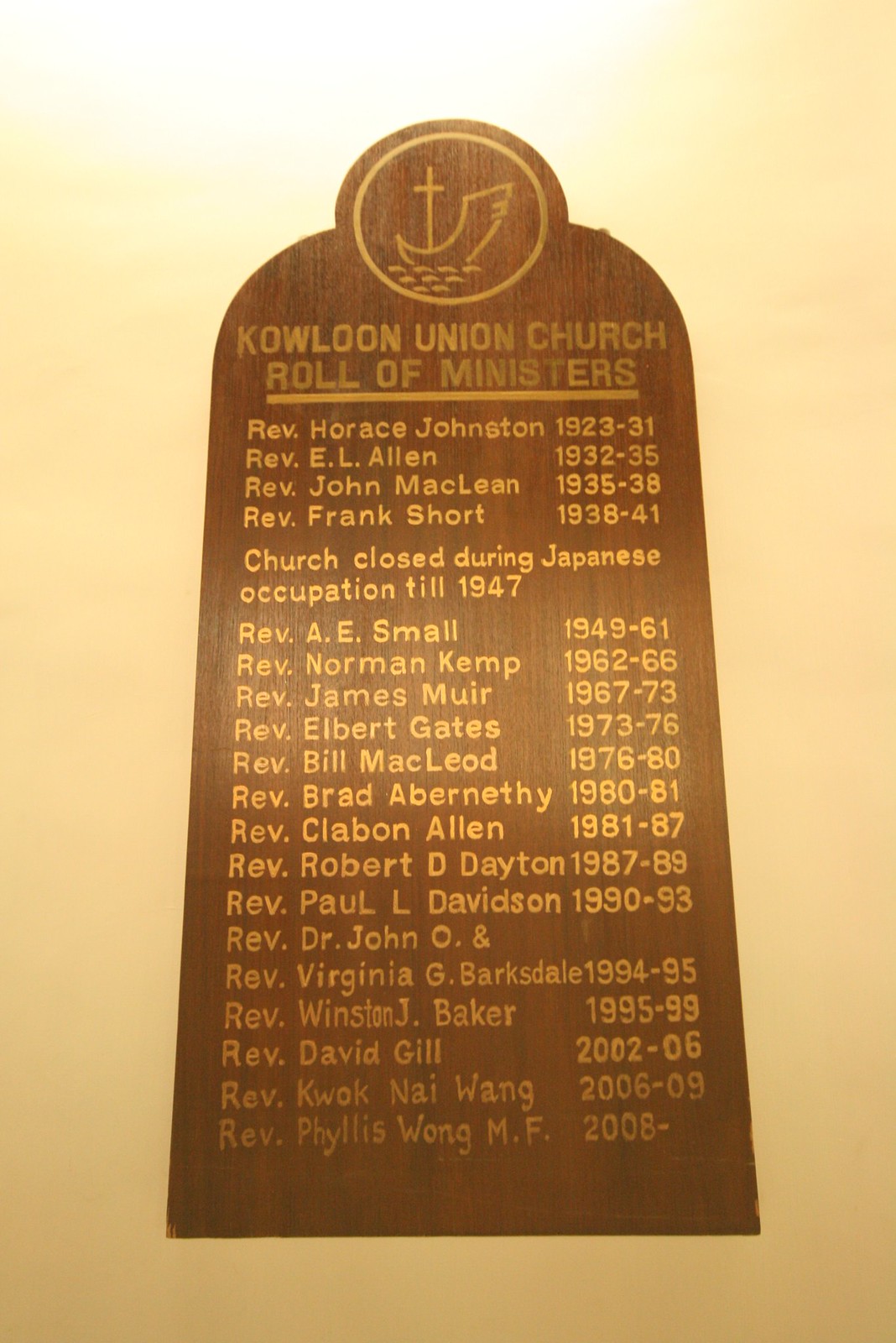The image showcases a wooden plaque affixed to the wall indoors, likely within a church setting. The plaque, which resembles a round cathedral window, features a circular top section displaying a logo depicting a boat with a cross on water. Below this logo, gold lettering reads "Kowloon Union Church Roll of Ministers." This plaque commemorates the ministers who have served at the Union Church, listing their names and service years. Notably, it begins with Reverend Horace Johnston (1923-1931) and proceeds through a detailed timeline, including Reverend E.L. Allen (1932-1941), Reverend John McClain (1935-1938), and many others, noting a closure during the Japanese Occupation until 1947. The list continues with ministers like Reverend A.E. Small (1949-1961), Norman Kemp, James Muir, Elbert Gates, and Reverend Bill McCloud, among others. The most recent entry is Reverend Phyllis Wong, M.F., who has been serving since 2008 and is marked with no end date indicating she is the current minister. The names and dates are meticulously handwritten in gold on the wooden background, emphasizing the historical continuity of the church's leadership.